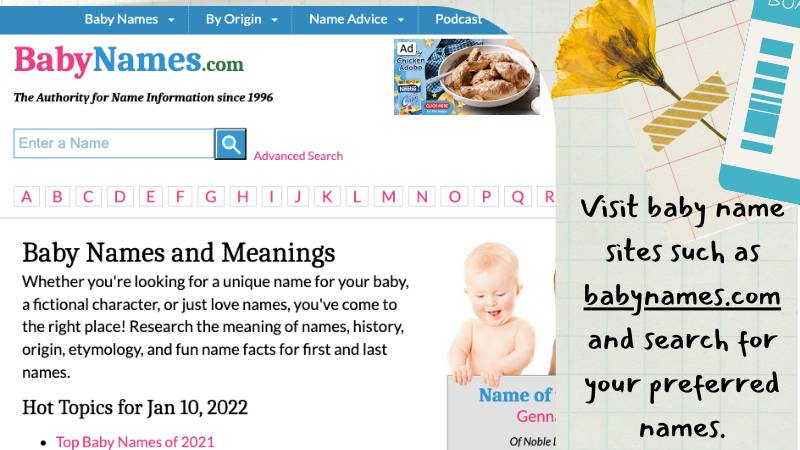This is a screenshot taken from the website babynames.com. At the top of the image, the navigation menu includes sections labeled "Baby Names," "By Origin," "Name Advice," and "Podcast." The page design gives the appearance of being partially peeled back on the right side, revealing a floral graphic and a card resembling a credit card. Text beside this visual reads, "Visit baby name sites such as babynames.com and search for your preferred names."

The website's name is prominently displayed on the top right, with "baby" in pink, "names" in blue, and ".com" in green. Beneath it, a tagline states, "The authority for name information since 1996." Below this is a search bar for entering a name, followed by a button labeled "Advanced Search" in pink.

As you scroll down, the alphabet appears across the screen starting with a pink letter "A" on the left, followed by "B," "C," "D," and continuing sequentially through to "Q" and "R" before being cut off by another image at the top. Further down, the site features sections titled "Baby Names and Meanings," "Hot Topics for January 10th, 2022," and "Top Baby Names of 2021."